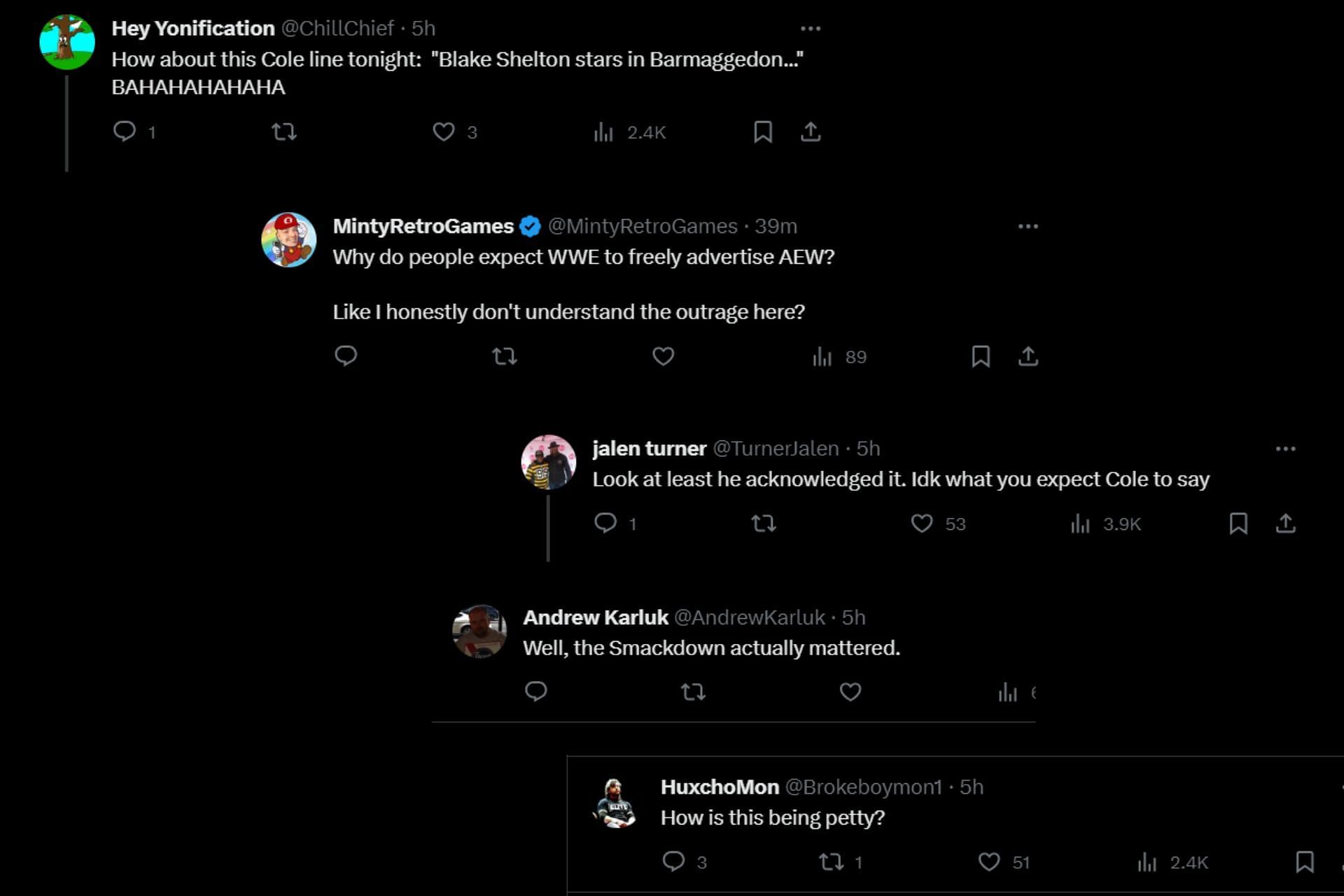**Descriptive Caption:**

A screenshot captures a lively discussion thread on the X (formerly Twitter) platform. The background is a solid black, emphasizing the text-based conversations. At the top of the screen is a post by "HeyYunification," humorously commenting, "How about this cold line tonight? Blake Shelton stars in Barmageddon. Ba ha ha ha ha," which has garnered 1 comment, 3 likes, and over 2,000 interactions.

The first reply, from "MintyRetroGames," questions, "Why do people expect WWE to freely advertise AEW? Like I honestly don't understand the outrage here," receiving 69 reactions.

Following this, "Jalen Turner" adds to the thread, "Look at least he acknowledges, I don't know what you expect Cole to say," earning 1 comment, 53 likes, and over 3.9 thousand interactions.

"Andrew Karlik" replies with his viewpoint, "Well Smackdown actually mattered," contributing further to the discussion.

Finally, "Huxo Mon" wraps up the thread with the comment, "How's this being petty?" highlighting the ongoing debate.

This image is illustrative of the vibrant and sometimes contentious discussions that occur on social media platforms.